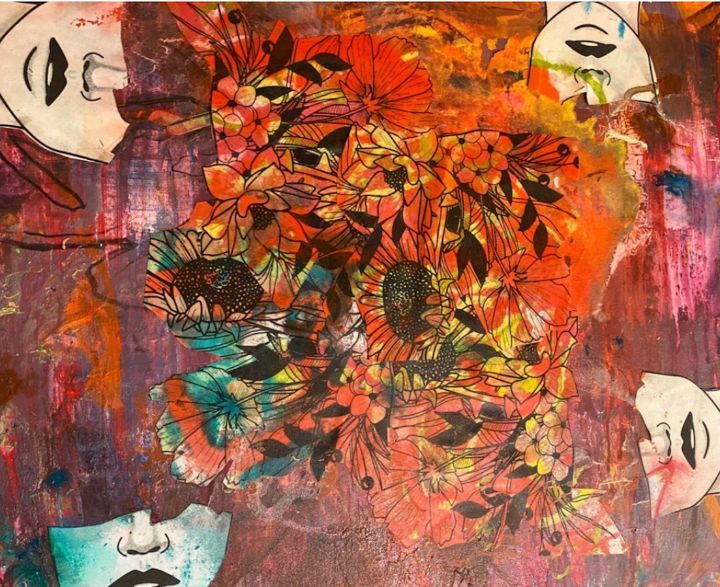The artwork is an abstract, mixed-media piece characterized by fine pen lines and various brushstroke techniques. Dominated by a chaotic array of sunflowers, the painting features dynamic red, orange, yellow, green, and orange-yellow hues. In the center, orange and multi-colored flowers, resembling black-eyed Susans with dark centers, blend into a vibrant background of purple, orange, blue, and white streaks. Surrounding the central floral cluster are four half-faces, each representing the bottom part of a face from the nose downward, with distinct dark lips. These faces are oriented differently in each corner: one face is upright in the bottom left, another is sideways on the right, a third is upside down in the top right, and the last is sideways on the left. Each face also exhibits different colored marks, including blue, green, and red, adding to the intricate and chaotic details of the artwork.